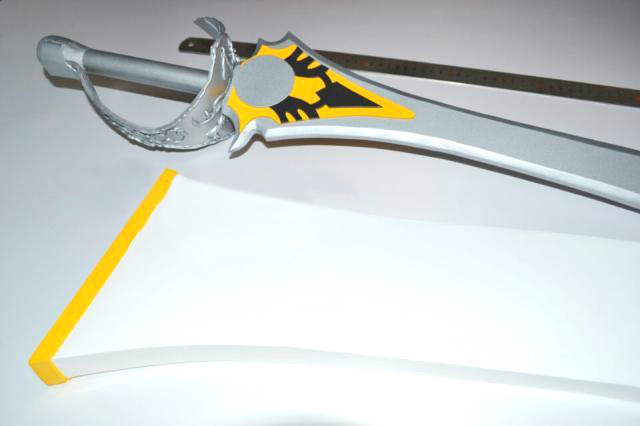The image is a close-up of a toy sword laid on a flat, likely wrinkled white surface. Positioned next to the sword, to its right, is what seems to be its scabbard. Additionally, a partially visible metallic, reflective ruler with a hole on the left and marked with numbers and notches is present at the top. The toy sword, featuring a round basket-type hilt and a thick, dull blade, is primarily silver in color with yellow detailing on the blade. The scabbard, also silver, displays a yellow and black symbol with a silver circle at the top. The overall arrangement is horizontal, with the toy sword centrally placed, the ruler partially covering it from above, and the scabbard beneath it. The background appears light gray to white, emphasizing the toys and tools against the surface that may suggest a domestic or curated setting.